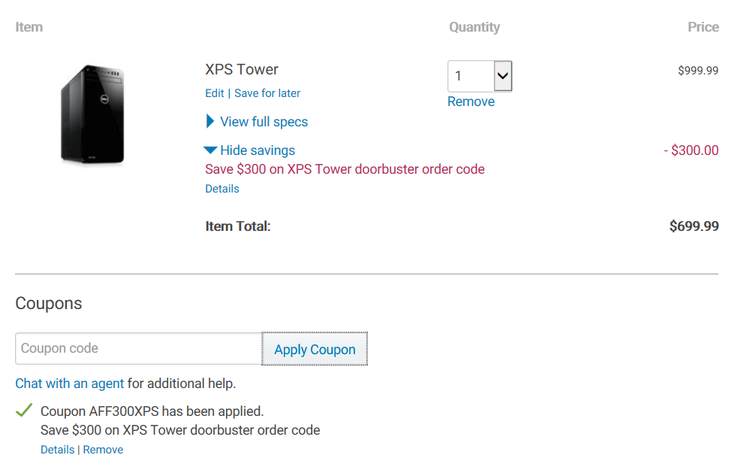This screenshot shows a cropped section of a webpage displaying details of an electronic product purchase. The item in focus is a black computer tower labeled "XPS Tower." Below the item title, there are two interactive buttons: "Edit" and "Save for Later." Underneath these buttons, there are options labeled "View Full Specs" and "Hide Savings," each accompanied by a small arrow indicating that more information can be revealed by clicking them. 

The "Hide Savings" option is selected, displaying a promotional offer in maroon text: "Save $300 on XPS Tower Door Buster Order Code." Below this, "Details" is indicated in blue text. The item total before the discount is shown at the bottom in bold black font.

On the right side of the screenshot, the original price of the XPS Tower, $999.99, is listed. Directly below this, in maroon text, the $300 deduction is noted, bringing the final order total to $699.99, which is prominently displayed in bold black font. 

At the bottom of the screenshot lies a horizontal line separating this section from the coupon code input area. Here, there is a text box to enter a coupon code with an "Apply Coupon" button next to it. Additionally, there is a prompt offering the option to chat with an agent for further assistance. The user appears to have already entered the code referenced in the promotional offer.